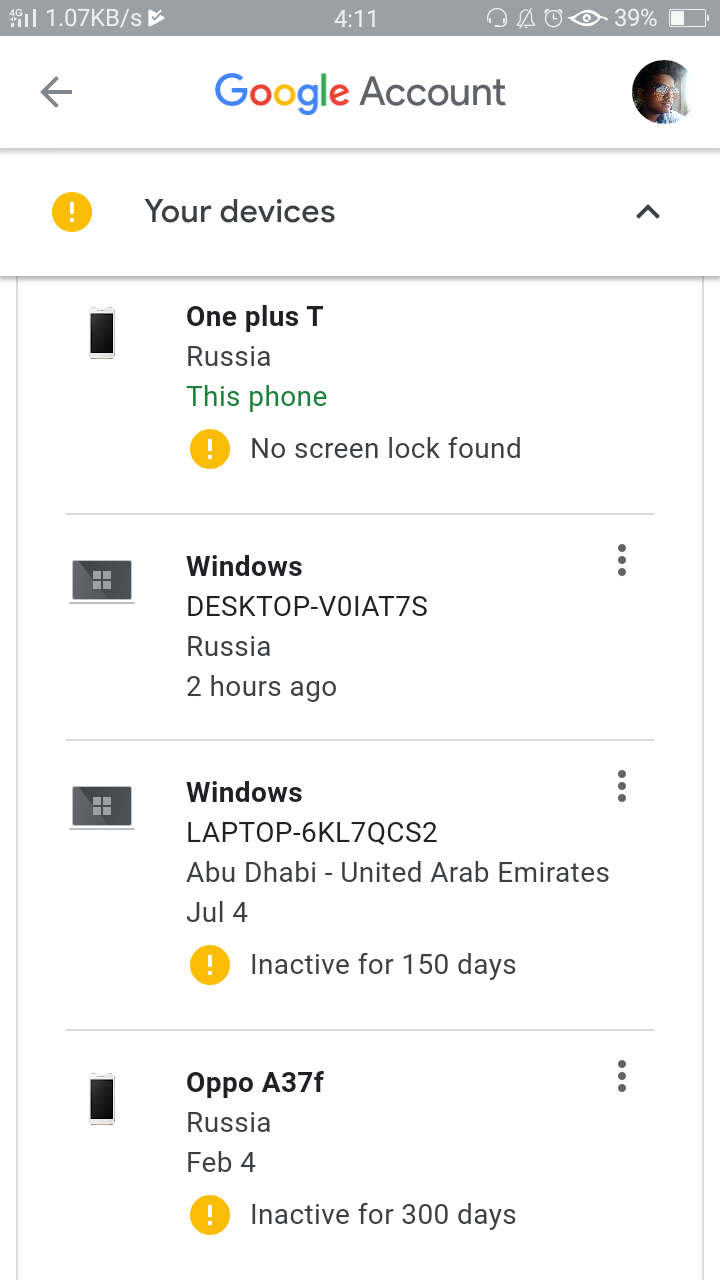This is a detailed screenshot from an Android device, potentially a Samsung phone. At the top of the image, a gray status bar is visible, indicating a 4G connection with full signal strength. A small display shows data usage at 1.0 KB/s alongside a playing icon, suggesting ongoing activity.

In the center of the status bar, the time reads 4:11. Various icons are clearly visible: a pair of headphones, a bell, a clock, and a leaf symbol. The battery icon shows a 39% charge level.

Just below the status bar on the left side, there is a circular icon containing a quotation mark, labeled "Your Devices." To the right, an upward-pointing arrow is present. The main section of the screenshot is divided into four distinct areas:

1. **OnePlus T (This Phone)**: On the left, a circle with an exclamation mark indicates that no screen lock is found. The right side displays an icon resembling a phone.
2. **Windows Desktop (Voit7s)**: Labeled as a device located in Russia with activity noted from two hours ago, indicated by a laptop icon on the left and accompanied by three dots representing additional options.
3. **Windows (Laptop)**: Featuring a laptop icon, it shows detailed information, likely including model specifics.
4. **OPPO (Phone)**: Another device listed as being in Russia, this phone has been inactive for 300 days, marked with a circle and an exclamation mark icon.

Each section represents a different device and provides connection or activity status, enhancing the organizational clarity of the information on the mobile device.